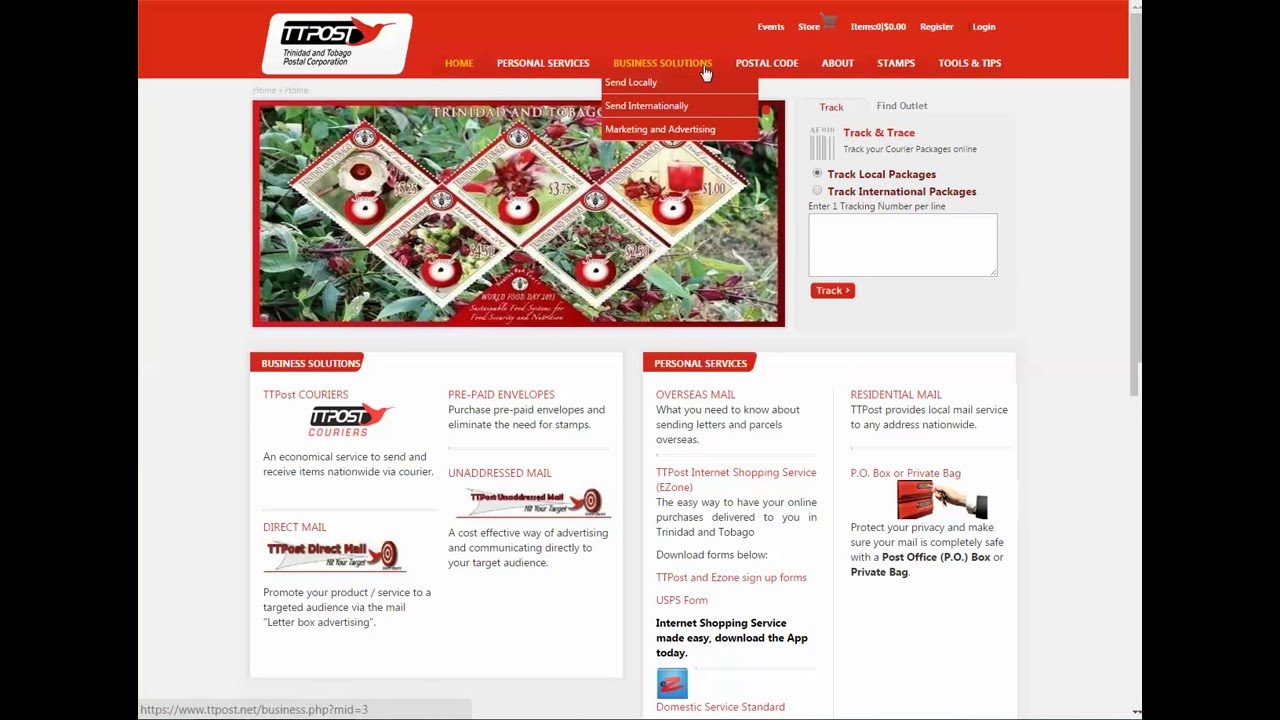The image showcases the T.T. Post website, set against a pitch-black background, making the site itself stand out prominently. At the top of the website, there's a striking red banner. To the left of this banner is the T.T. Post logo, which features a white rectangle background with the text "T.T. Post" accompanied by a red bird icon. The text within the logo is set against a black background, accompanied by some hard-to-read subtext beneath it in a bright shade of flesh color.

To the right of the logo, the navigation bar prominently displays links titled "Home," "Personal Services," "Business Solutions," "Postal Code," "About," "Stamps," "Tools and Tips." The upper portion of the page also includes sections labeled "Event Store" and some additional, less legible information.

On the left side of the website, there appears to be an image displaying a pattern of squares arranged in the shape of a 'W'. Each square contains a circular design with a red outline, a white center, and a black dot within it.

Below this image section, there are various headings and details about services offered by T.T. Post. The "Business Solutions" section mentions T.T. Post Carriers along with relevant information. Similarly, the "Personal Services" section provides details on services like overseas mail and residential mail, helping users understand the range of offerings available.

Overall, the T.T. Post website is well-structured with a clear emphasis on its services and navigation, despite some elements being difficult to read.